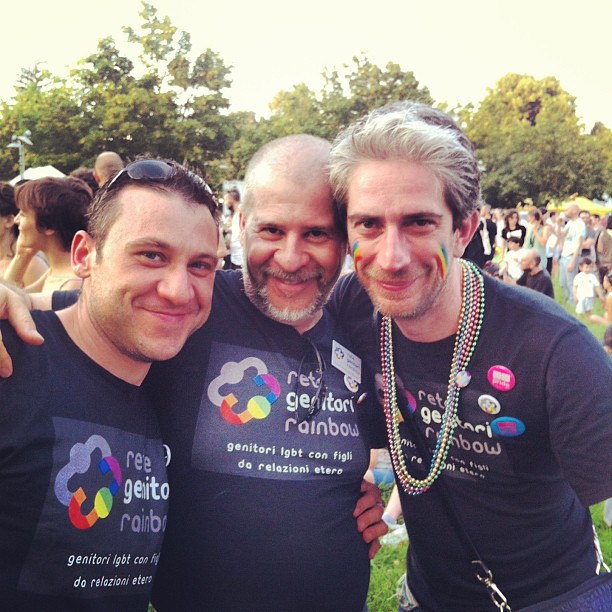In this vibrant outdoor photo taken at a likely gay pride festival, three smiling men are huddled together, taking a selfie and showing strong support for each other. Each man is wearing a dark T-shirt that reads, "Rete Genitori Rainbow Genitori LGBT Con Figli," adorned with a rainbow and a chain-link design, partially obscured by wrinkles. The man on the left, who appears to be in his 30s or early 40s, has short hair and sunglasses perched on his head. The man in the middle, possibly in his 50s, has a bald head and sports a gray beard and mustache, with a pair of sunglasses hanging from his shirt. The man on the right, also in his 50s, has whitish-gray hair, a stubbly beard, and is decorated with rainbow face paint on both cheeks as well as colorful beaded necklaces reminiscent of Mardi Gras beads. Behind them, a large crowd is visible, mingling in what seems to be a grassy, tree-lined area under the open sky. The image captures the essence of joy, solidarity, and celebration within an LGBT community event.